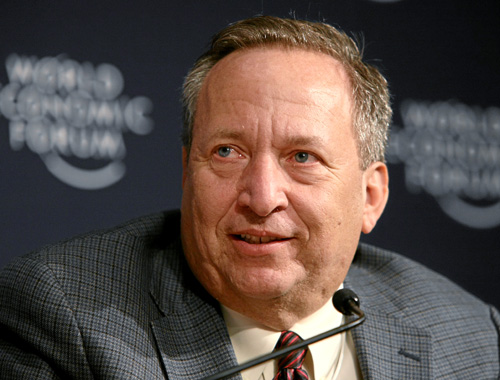This is a photograph of Larry Summers at the World Economic Forum. Larry Summers, an economist and the former president of Harvard University, is also known for his service in the Clinton administration. He is dressed in a checkered suit paired with a red and black striped tie and a white shirt. A black microphone is positioned directly in front of him as he looks to his right, with his short hair parted on the side, and sporting a slight smile. The background features a blue wall with the text "World Economic Forum" repeated at least twice, suggesting it continues across the entire wall. The colors in the image include shades of brown, black, white, silver, and tan for his skin. The photo appears to be slightly wider than it is tall, and Larry Summers may be either seated or standing, as the photograph is cropped and does not provide a clear indication of his position. The setting is indeterminate regarding whether it is indoors or outdoors, or if the photo was taken during the day or at night.